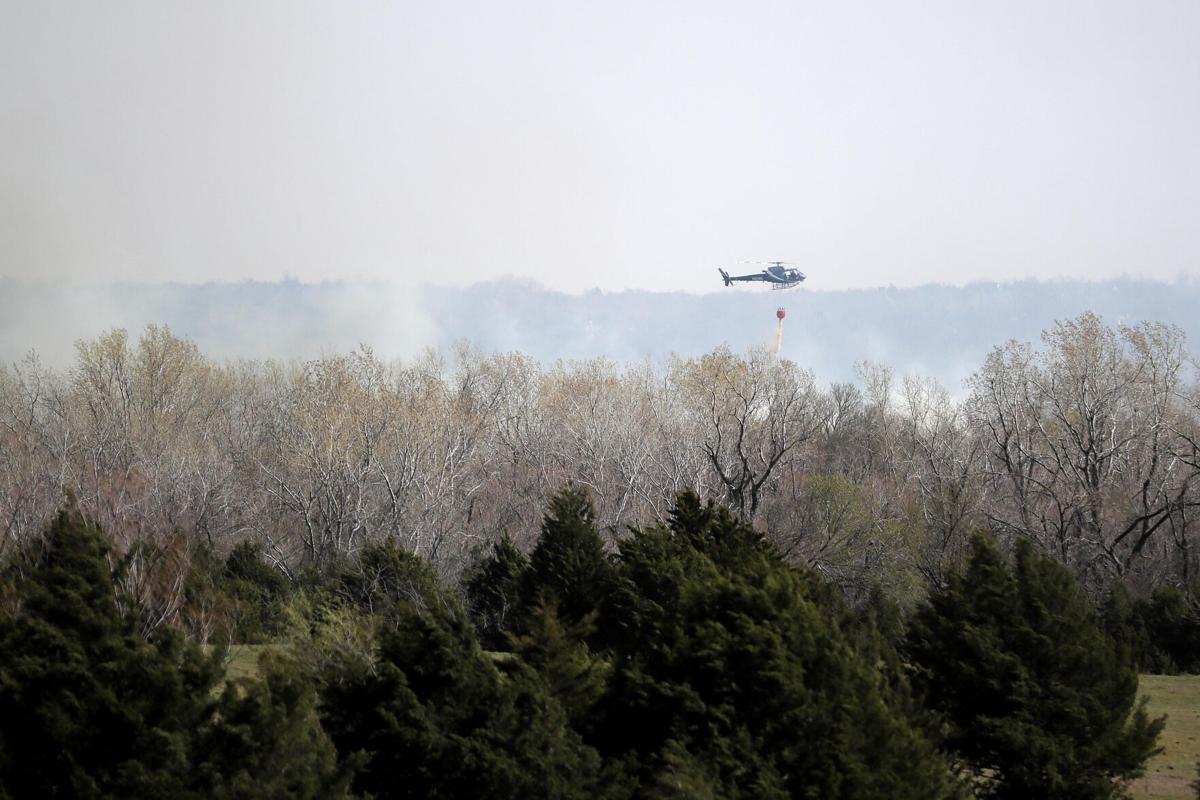This is a horizontally aligned rectangular photograph taken outdoors during the daytime. Dominating the center-right portion of the image, a gray or blue rescue helicopter is flying towards the right, with a large red and yellow rope or orange bucket hanging down from it, and water cascading out in a light brown stream. The helicopter appears to be engaged in firefighting efforts over a forest fire, which is suggested by the gray smoke billowing upwards from the midsection of the image.

The upper portion of the picture is filled with a cloudy, light grayish sky, tinged with smoke that has blurred the finer details. Just below this sky, a subtle outline of barren deciduous trees without leaves is visible, extending horizontally across the image. These trees stand in stark contrast to the vibrant greenery present in the foreground.

In the lower half of the picture, a row of dense, bright green pine trees contrasts with the barren branches above. Further down, closer to the base of the photograph, taller pine trees dominate the scene, their green canopies adding a lush element to the composition. Additional detail on the right and a little on the left shows a hill with green grass, further framing the action occurring in this snapshot of a firefighting operation in progress.